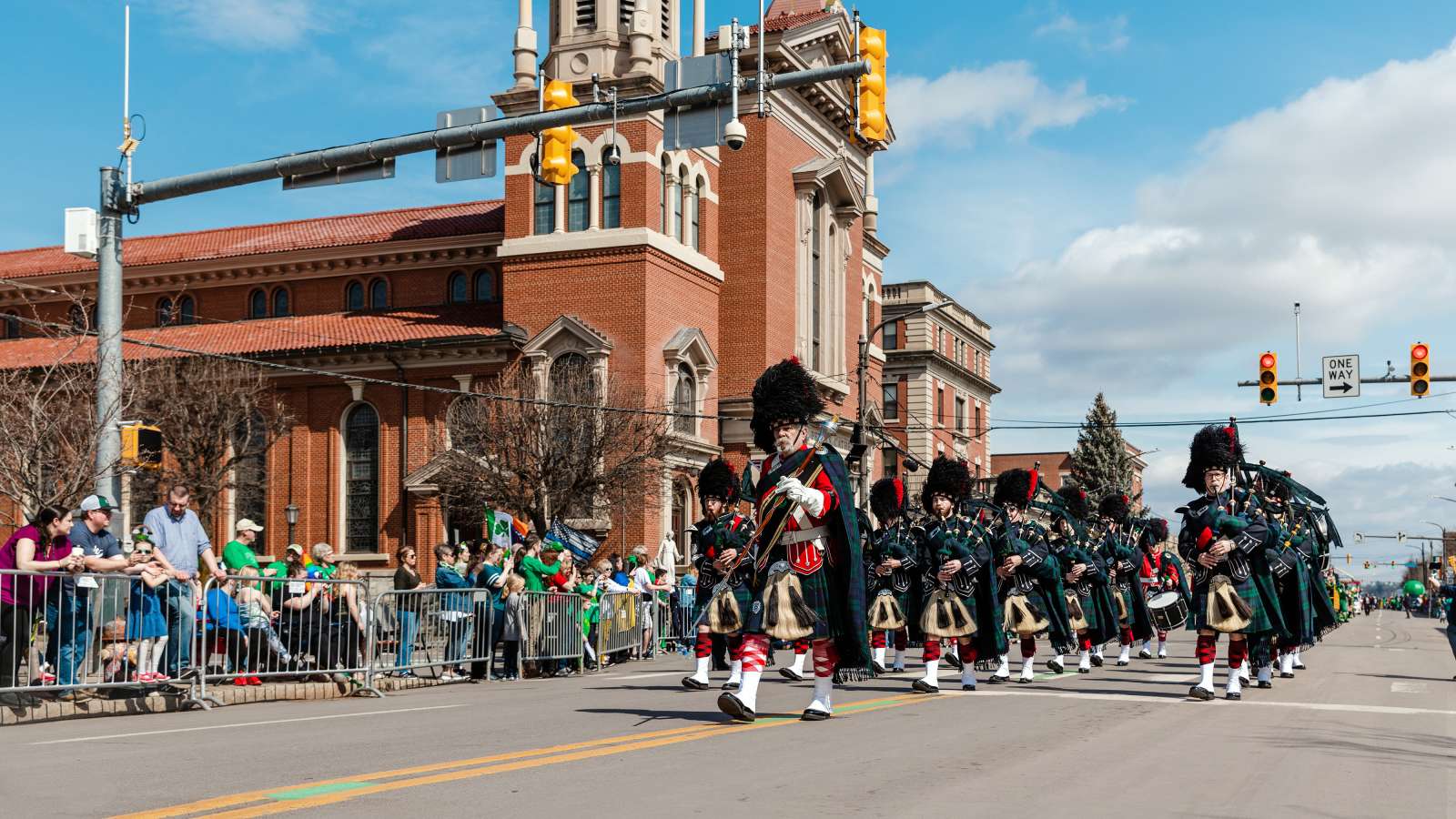The image captures a festive parade making its way through the heart of a small town, viewed from a low angle. The focal point is a leading bagpiper dressed in a traditional Scottish uniform, distinguished by a black fur hat, a long black coat, a kilt, and white boots, while carrying his bagpipe across his shoulder. Following him are three lines of identically dressed bagpipers, actively playing their instruments. The parade route is lined with silver metal barricades, behind which spectators are seated or leaning over to watch the event. A clear, sunny day with scattered clouds sets a cheerful backdrop. In the upper left, the facade of a red brick cathedral with white-outlined arched windows and a terracotta roof is visible. To the upper right, a red traffic light shines above a "One Way" sign. The street is entirely closed off for the parade, ensuring an uninterrupted celebration for both the participants and the onlookers.